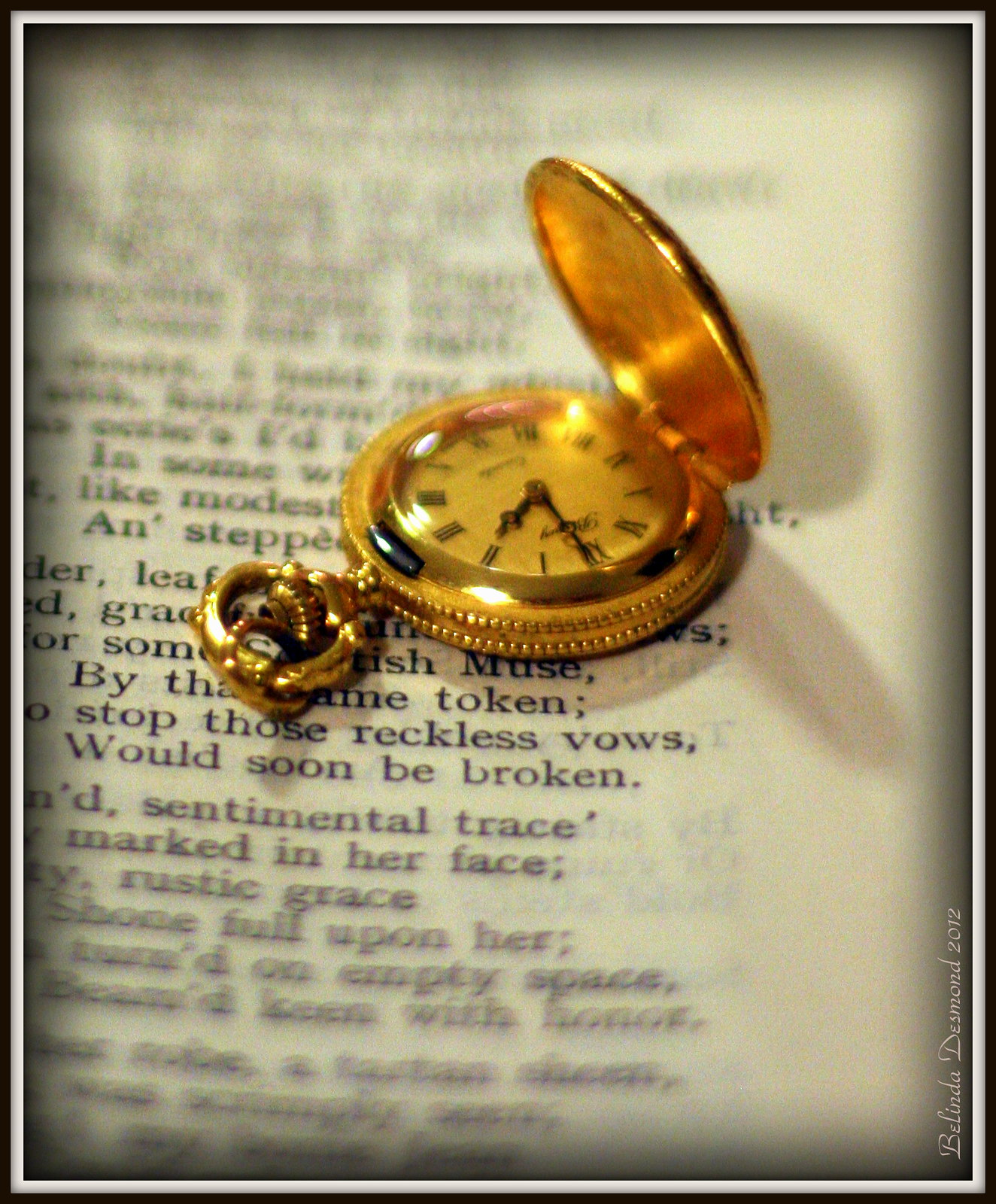The image showcases a gold wind-up pocket watch, approximately double the size of a silver dollar, lying on a piece of white paper with black printed text. The pocket watch, which prominently features a cover that must be opened to view the time, displays Roman numerals and indicates a time around 8:30 to 8:31. The watch has no wristband, aligning with its classification as a pocket watch. The text on the paper is largely unreadable and uninteresting, yet a discernible fragment reads, "stop those reckless vows, you would soon be broken." The watch casts a shadow on the paper, which reinforces its flat positioning atop the surface. The sharpness of the paper's text is insufficient to allow for any additional clarity.